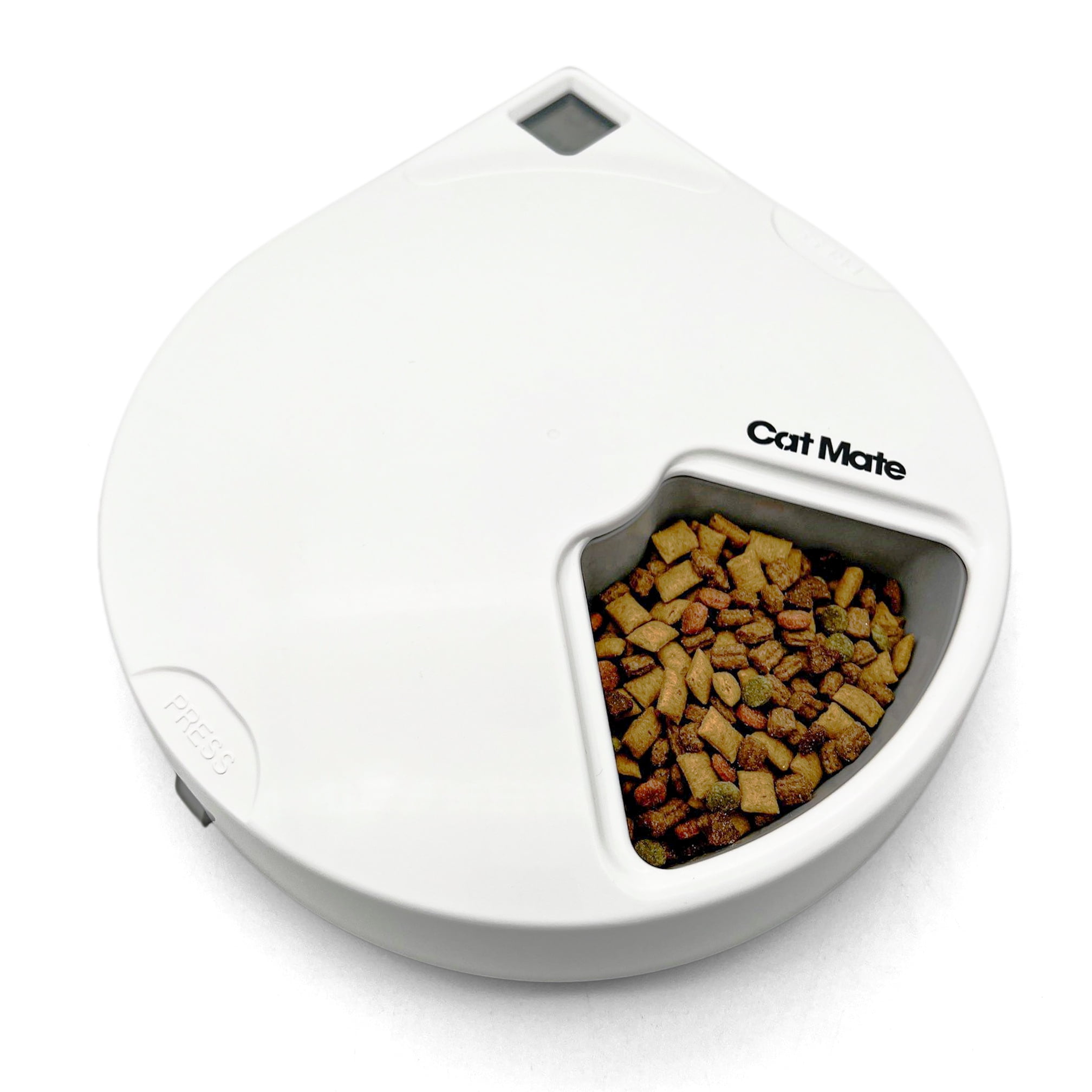This full-color promotional photograph showcases a Cat Mate, an automatic food dispenser for cats. The device features a round, white plastic base with flat walls on the sides. It has a triangular-shaped opening in the front, curved at the top and rounded at the bottom, with black text reading "Cat Mate." Inside this opening, a dish filled with regular cat food, comprising shades of brown and light green, is visible. In the lower left-hand corner is an indented area with raised lettering that says "PRESS." The upper right-hand corner of the device includes a squared-off section housing a small, gray digital display used for programming the feeding schedule. A subtle shadow beneath the device on the white background adds depth to the image. The Cat Mate's programmable rotating bins and selective openings ensure scheduled feeding, allowing you to monitor and manage your pet's eating habits even when you're away.